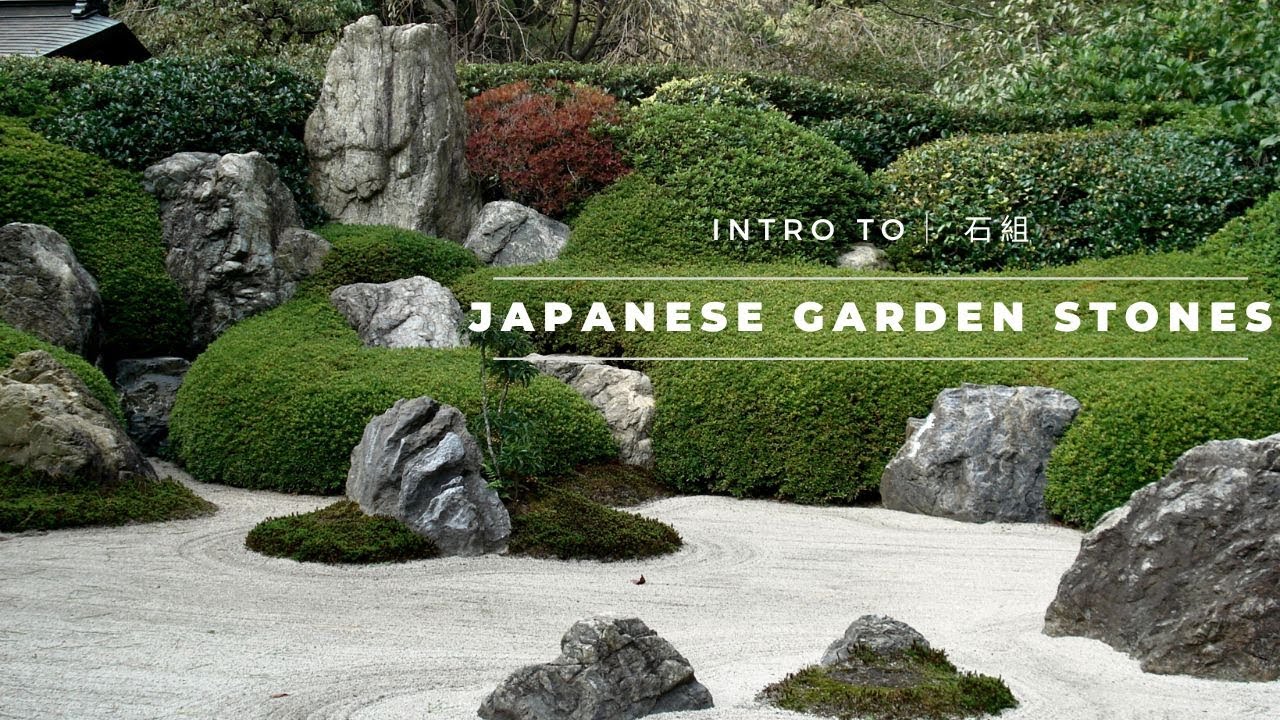The image depicts a meticulously maintained Japanese garden, prominently featuring the text "Intro 2" in bold white capital letters at the center. Adjacent to this title are characters in an Asian script, followed by another line of text that reads "Japanese Garden Stones," also in white. This caption is enclosed by thin white lines above and below. The garden itself showcases a serene blend of natural elements, with large, hefty boulders scattered across an orderly raked dirt area, forming perfect circles and lines around each stone. 

In the foreground, two substantial stones are visible, one adorned with a patch of green grass. The middle and upper left portions of the image are dotted with clusters of stones interspersed with lush green grass. The scene is further enriched with a burgundy bush and what appears to be a bridge or pathway in the upper left corner. On the right side, hedges frame the composition, adding to the sense of natural harmony. Toward the bottom of the image, there is freshly raked white sand surrounding gray and white rocks. Accompanying this tranquil setting, gray swirly water can be seen, blending seamlessly with the boulders and greenery. The overall effect is a perfect balance of stone, greenery, and carefully crafted sand patterns, offering a visual representation of a traditional Japanese garden.